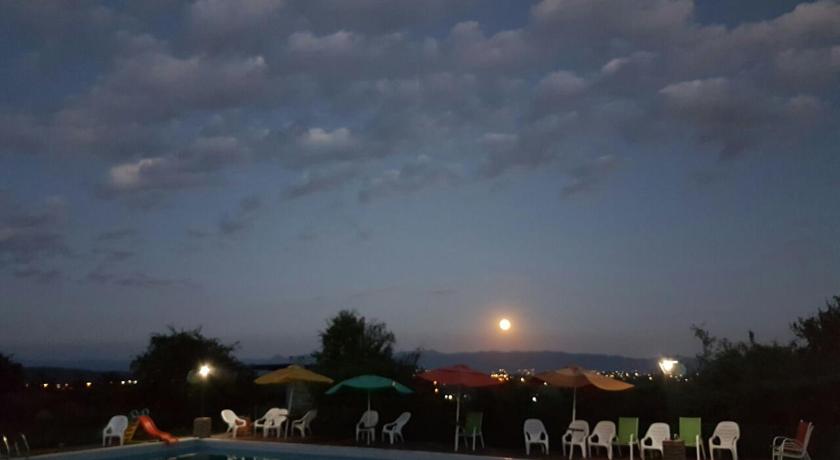This photograph captures a stunning scene of a sunrise taken from a high vantage point, possibly atop a mountain. The sky is dark, indicating early morning, with the sun emerging over a distant mountain range, casting a warm yellow hue across the horizon. Dark gray and white clouds punctuate the expansive sky, which has shades of blue blending with the dawn light. Below, a large swimming pool is surrounded by numerous white and green plastic patio chairs, hinting at leisure and relaxation. The pool area is also adorned with big umbrellas in vibrant colors – yellow, light blue, red, and gold – adding a touch of brightness to the dimly lit morning. In the background, the silhouettes of trees and a hilly landscape emphasize the elevation and serene remoteness of the location. Lights from a distant city twinkle faintly, while the overall scene suggests a warm, inviting atmosphere, ideal for an early morning dip or quiet contemplation.